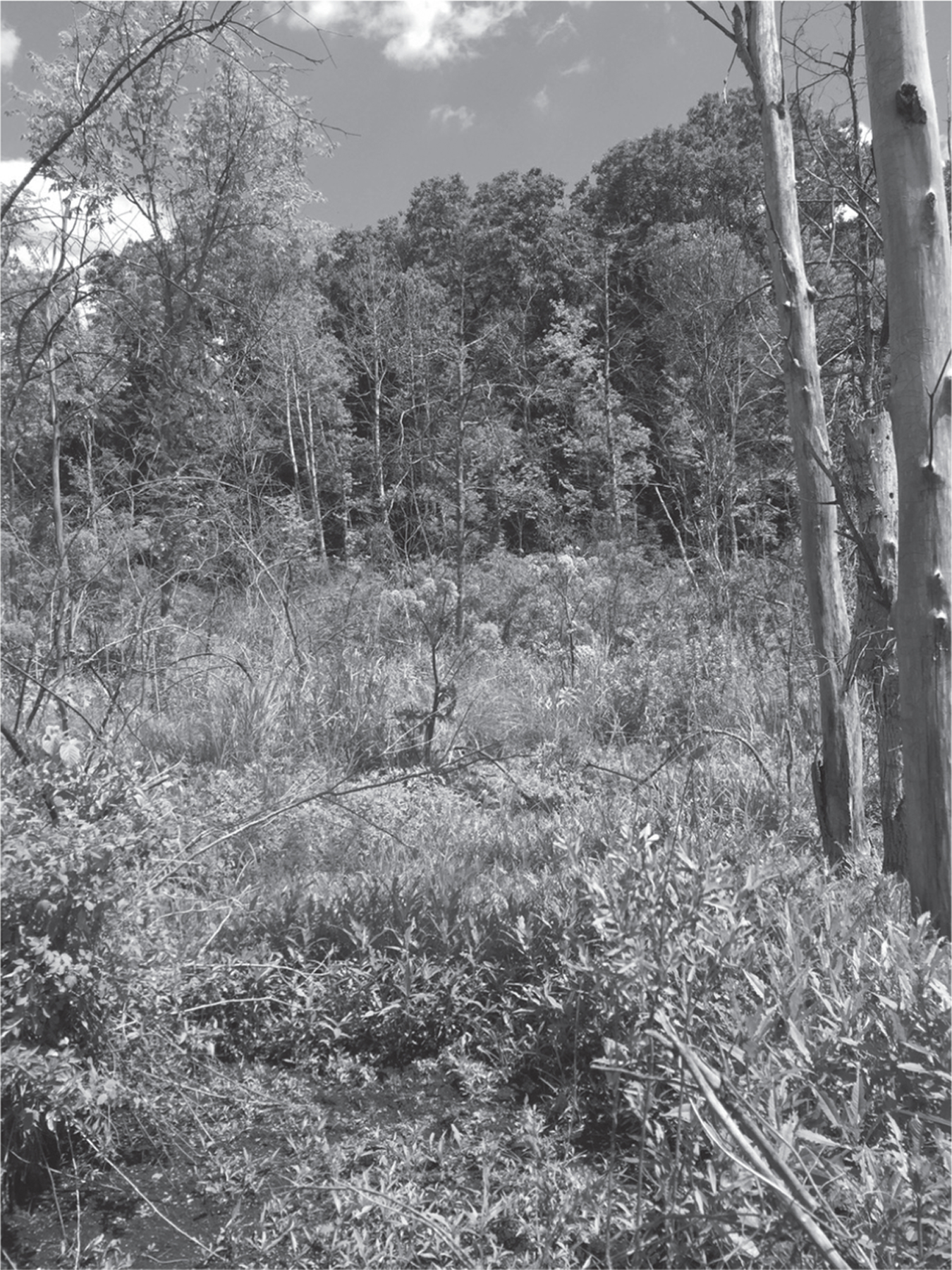This black-and-white photograph captures a forest scene with intricate details in various shades of gray. It appears to be midday, as the sunlight casts distinct shadows beneath the elements within the frame. The composition features a gentle hill rising towards the top, creating a dynamic perspective from the grassy foreground to the densely packed trees in the background. The foreground is covered in shorter grasses and bushes, as well as a few bare branches scattered around. On the right side, several dead tree trunks stand tall, stripped of their bark and devoid of any foliage. In contrast, the left side of the image showcases a mix of spindly, leafless trees and some taller, leafy ones, creating a stark juxtaposition. The sky, visible at the top of the image, is largely clear with a few wispy clouds and a puff of white on the far left. Throughout the image, the absence of coniferous trees and the predominance of deciduous ones contribute to the seasonal atmosphere, suggesting this scene is captured in the summertime. Despite the overall dense forest in the background, the varied tones of black, white, and gray bring out the contrasts and details within this somber, yet richly textured landscape.